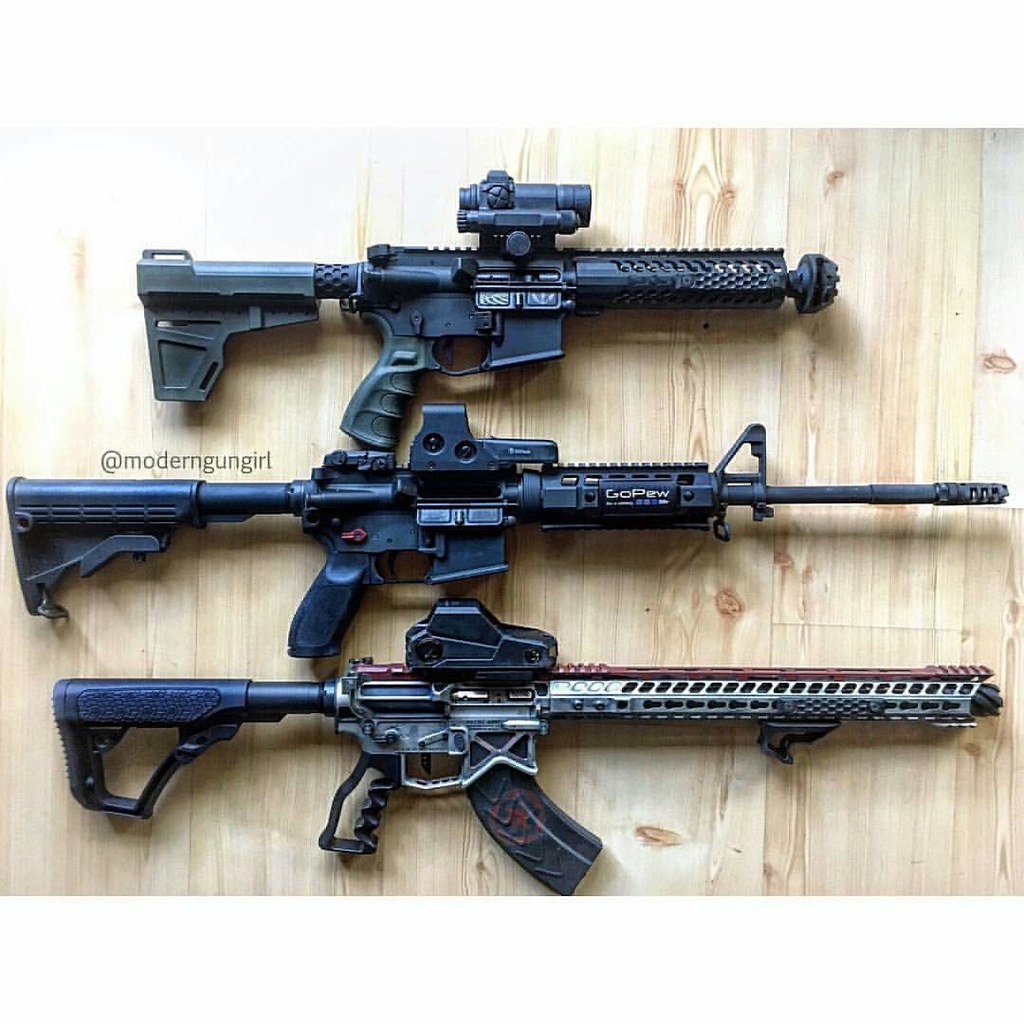This is a highly detailed color photograph of three rifles arranged vertically on a light wooden surface, all pointing towards the right side of the image. Each rifle differs in design and features, but they all share a sleek black color.

1. The rifle on the top features a short black barrel, a scope mounted on the top, a textured rubber grip, and a shoulder stock. It also has a green handle.
2. The middle rifle has a long, thin barrel with the word "GOPEW" inscribed on it. It boasts a smooth handle and an extended shoulder stock.
3. Positioned at the bottom, the rifle is distinguished by its very long barrel, which includes silver and red details. Similar to the others, it has an additional item bolted on top whose function is not immediately clear but is predominantly black in color. A shoulder stock extends from the back.

On the far left of the image, slightly above the middle rifle, the Twitter handle "@modern_gun_girl" is prominently displayed. The photograph is contained within a square frame, giving a balanced and organized appearance to the arrangement of the rifles. The combination of textual and visual details provides a comprehensive and precise depiction of the firearms and their positioning.